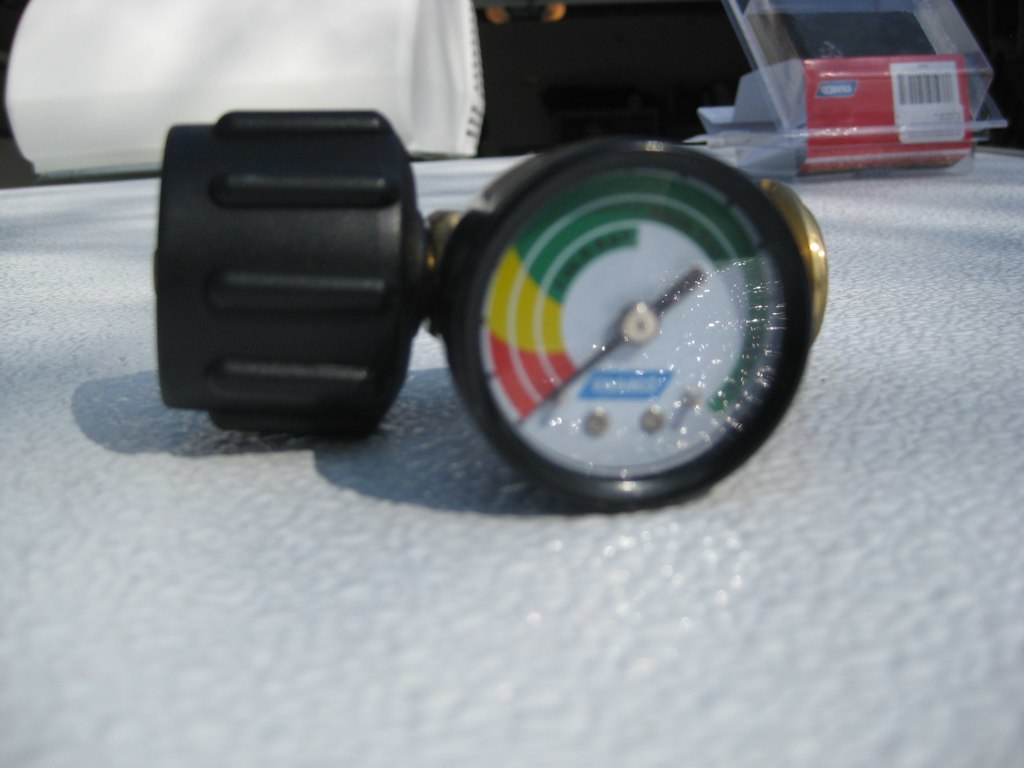A slightly blurry, landscape format photograph features a pressure gauge prominently in the foreground. The gauge appears to be sitting sideways on a white, bumpy surface and seems disconnected from any apparatus, such as a gas canister, to which it should be attached. Despite the blurriness of the gauge itself, the background is in higher resolution, though it contains no distinguishable features. The gauge dial is marked with color-coded sections: green for low, yellow for moderate, and red for high pressure. Interestingly, the needle is pointing to the high red section, likely indicating its default setting before being properly connected.